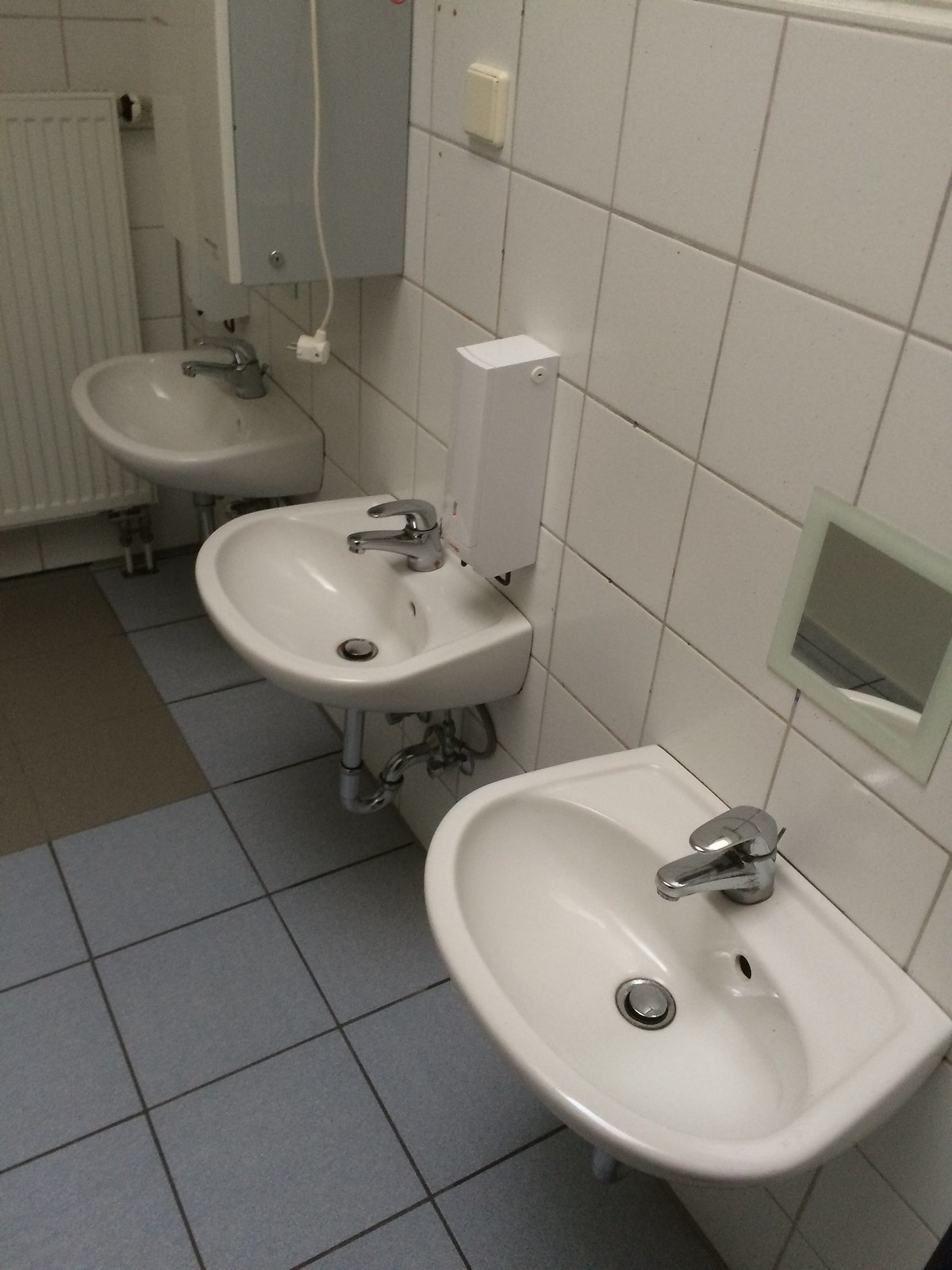This image captures the interior of a bathroom featuring a gray square-tiled floor with darker gray grout and some brown patches. The wall behind the sinks is adorned with smaller white square tiles. There are three identical white porcelain sinks, each equipped with chrome single-lever faucets and exposed chrome plumbing. 

The sink closest to the camera has a small, square-shaped mirror with a green border above it. The middle sink is topped by a rectangular white soap dispenser. The furthest sink from the camera features a cabinet above it, from which an extension cord hangs. Adjacent to this cabinet is a small, square beige button. On the wall adjacent to the sinks, there is a large, square-shaped radiator. A brown rug lies on the floor, adding contrast to the predominantly gray and white color scheme.

The bathroom appears to be photographed from a slightly elevated angle, offering a comprehensive view of the arrangement and elements present. The sinks seem lower to the ground, possibly indicating a setting catered to children, such as an elementary school.